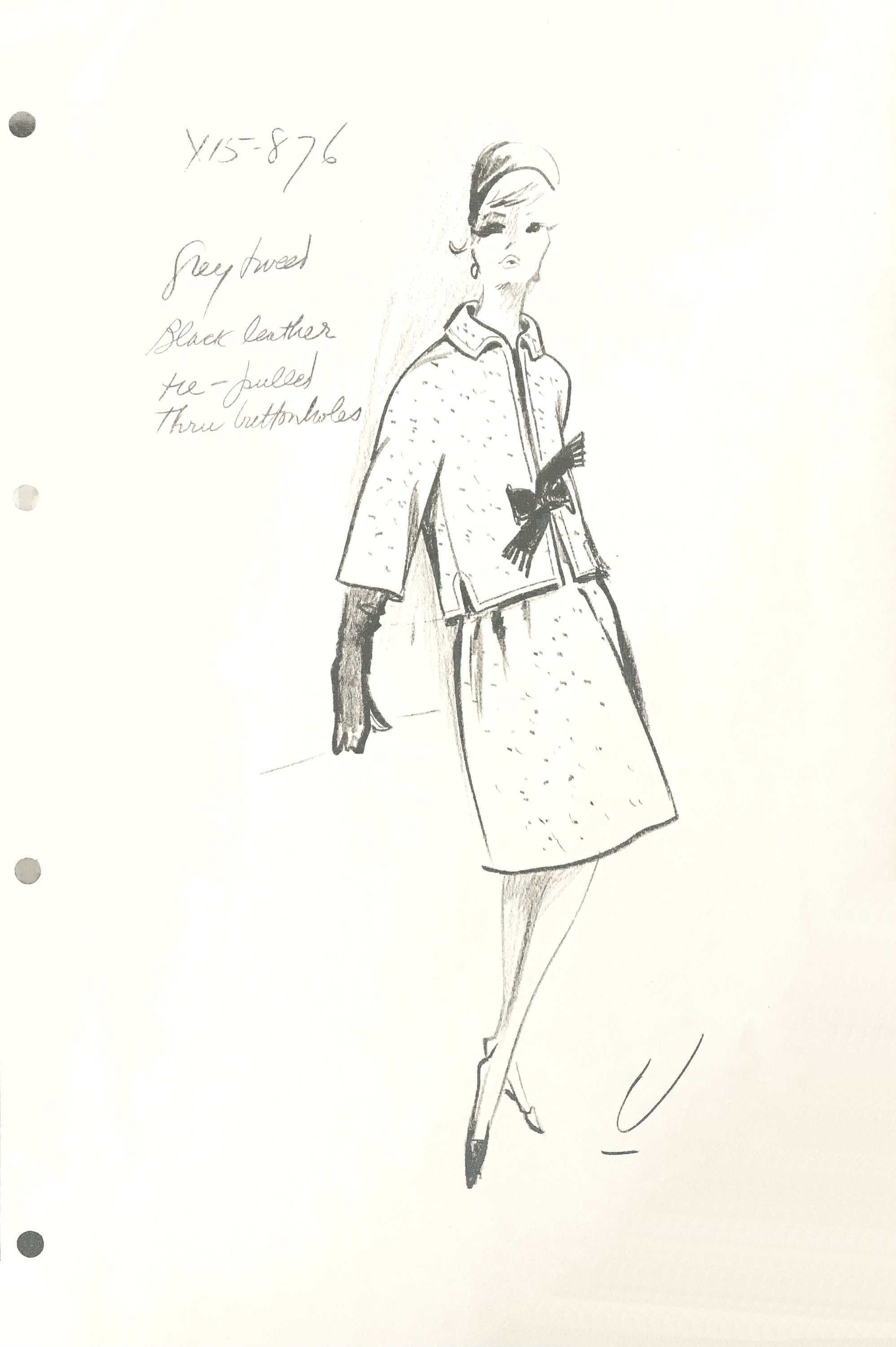This detailed black and white pencil sketch, possibly a scanned image, depicts a woman in a 1950s-style dress on a yellowed piece of ring binder paper. The binder holes on the left of the page appear as black circles due to the scanning process. The woman is fashionably dressed in a white top and white skirt with a dark ribbon tied just under the chest. She also wears black gloves and high heels, and her hair is styled in a bouffant. Her legs are crossed in a graceful pose, adding elegance to the sketch.

The dress includes a petticoat with detailed dotting, and she has a ribbon around her waist. At the top left of the image, the text "Y15-876" is prominently displayed, with additional but somewhat indistinct cursive writing underneath, possibly saying "gray treed, black leather, the pooled, three bottom holes." By her feet, the letter 'U' is underlined. The background of the paper has areas of gray shading, especially in the bottom right corner. There is also faint and unclear cursive writing at the top of the image. Overall, the meticulous detail in the sketch and the vintage style of the woman's attire are striking features of this artwork.